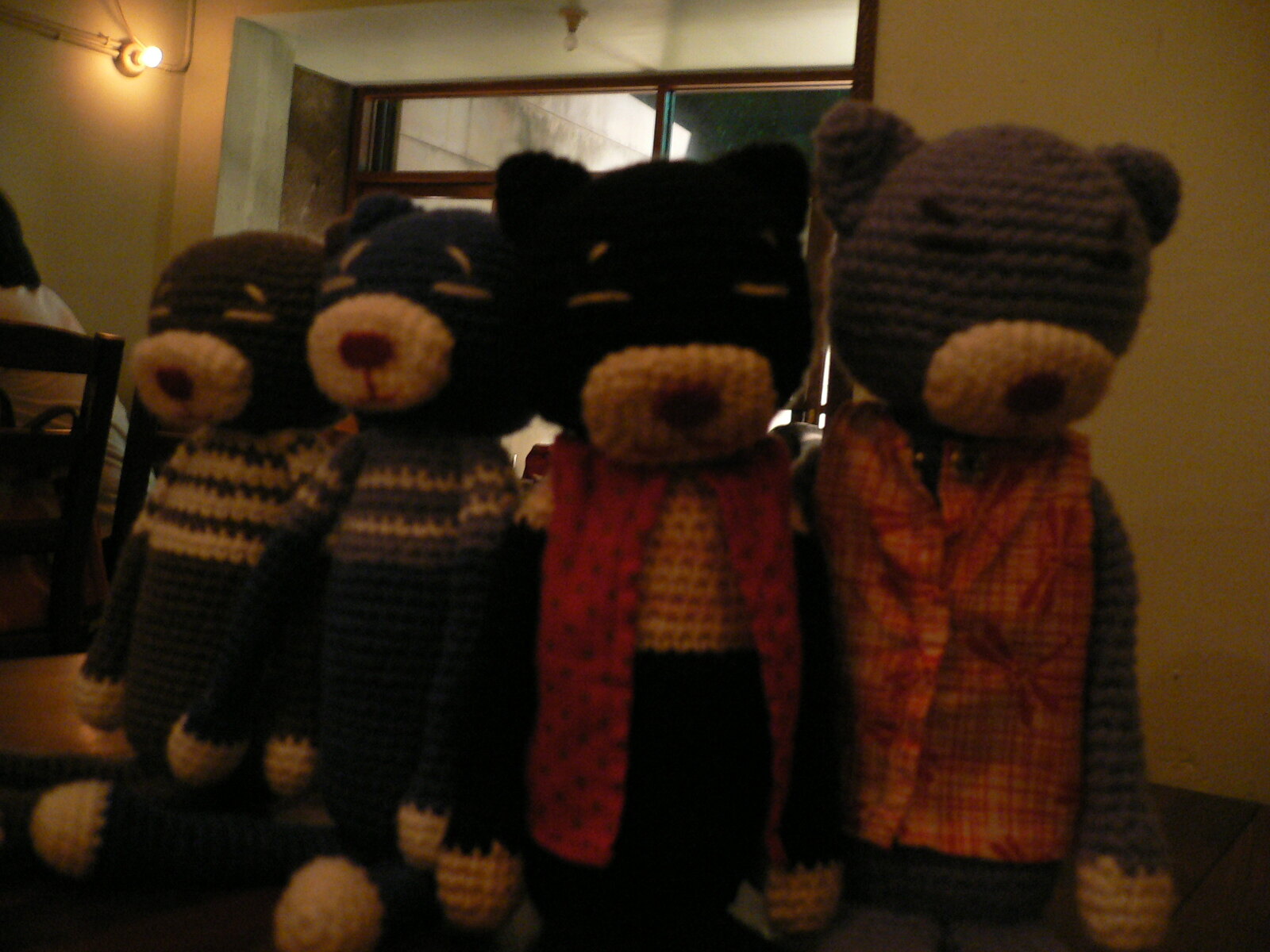The image captures four crocheted teddy bears seated in a row, each showcasing unique attire and a delightful array of colors. The bears, their eyes gently closed, appear to have been lovingly handmade. From left to right, the first bear is either a brown or gray color, dressed in an orange and red plaid shirt, its texture and hue somewhat indistinct due to the image's dim lighting. Next to it, the second bear stands out with its black and white coloring, complemented by a stylish red vest. The third bear is a soft light blue, adorned in a blue and white sweater that adds a cozy feel. Finally, the fourth bear, also light blue, sports a blue and white sweater, its design matching that of the third bear.

The setting seems to be a quaint restaurant or possibly a cozy home, as suggested by the wooden floors and a storefront-like door and window in the background. The ambiance is further warmed by the presence of exposed light bulbs on the wall, one brightly illuminating the scene. A glimpse of a person seated at a table can be seen to the left, adding a subtle touch of human presence to this charming tableau.